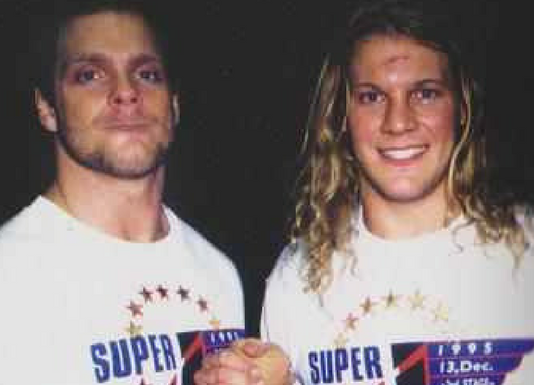This photograph captures a realistic and detailed close-up of two young individuals standing side-by-side, holding hands and depicted from the chest up. Both are wearing matching white t-shirts featuring a semicircle of gold stars on the front, with the text "SUPER" prominently displayed. Additional text on the shirts includes "1995" and "13 December," though the lower part of the text is partially obscured. The person on the left, who has short dark hair and a scruffy beard, has pursed lips. The person on the right has long, wavy blonde hair and is smiling, revealing their teeth. The background of the image is black, which highlights the two centered figures. The context suggests they are attending an event, possibly captured in a public setting by a photographer. The colors in the image include black, tan, brown, white, yellow, and red, further enhancing the detailed and expressive atmosphere.